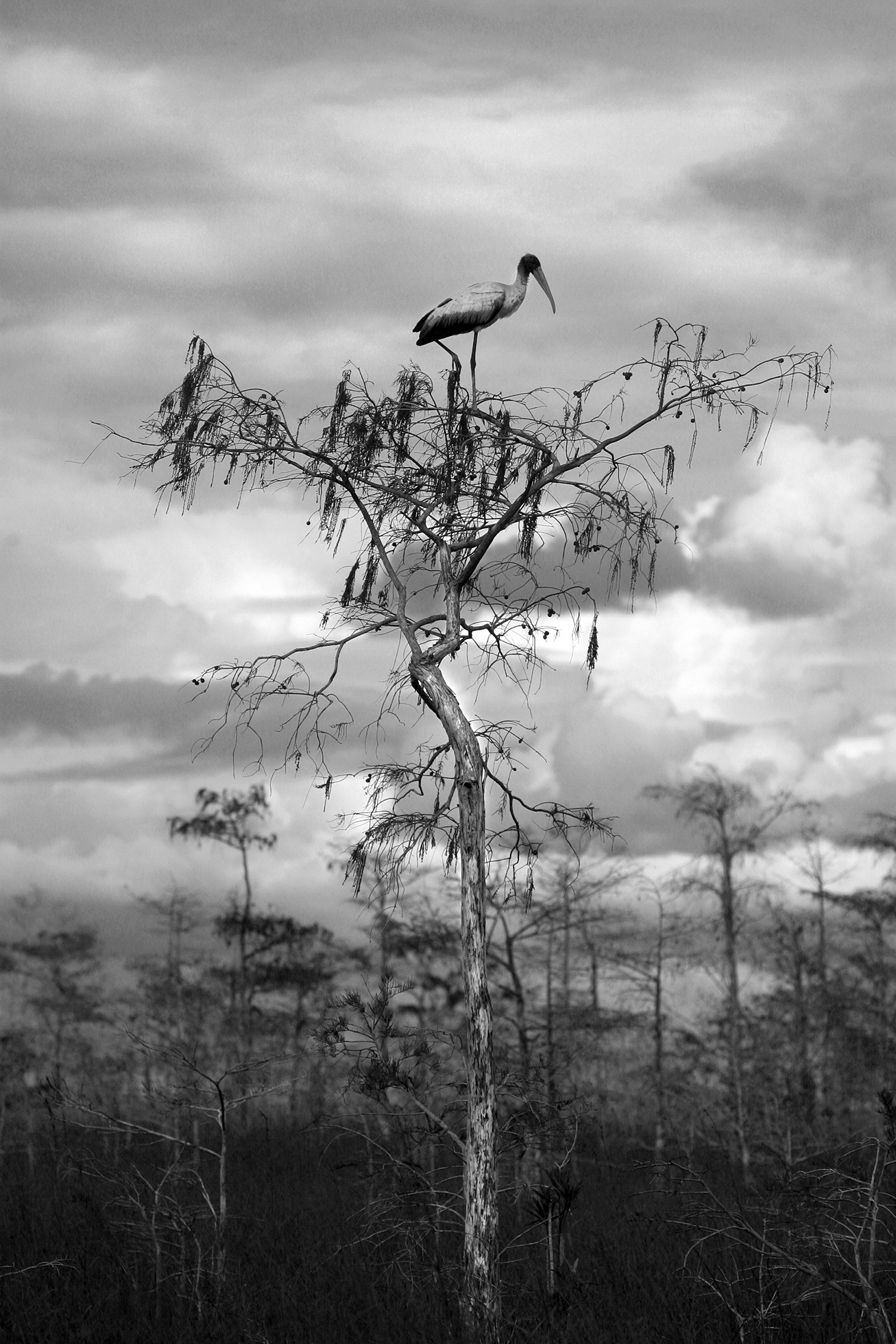This black-and-white photograph captures a hauntingly serene swamp scene under a cloudy, overcast sky. The very dark water at the bottom sets a somber tone, while the thinly foliaged trees lend an eerie, sparse beauty to the landscape. Front and center stands the focal point—a tall, scrawny tree with shabby, small branches and very few leaves. Atop this tree, a white bird with black-tipped wings and head perches delicately, clutching the branch with one foot while peering to the right. Surrounding this central tree are smaller, equally barren trees, adding to the desolate and mysterious ambiance of the image. The prominent gray clouds rolling across the sky heighten the photograph's brooding atmosphere, suggesting an impending storm or a lingering fog.